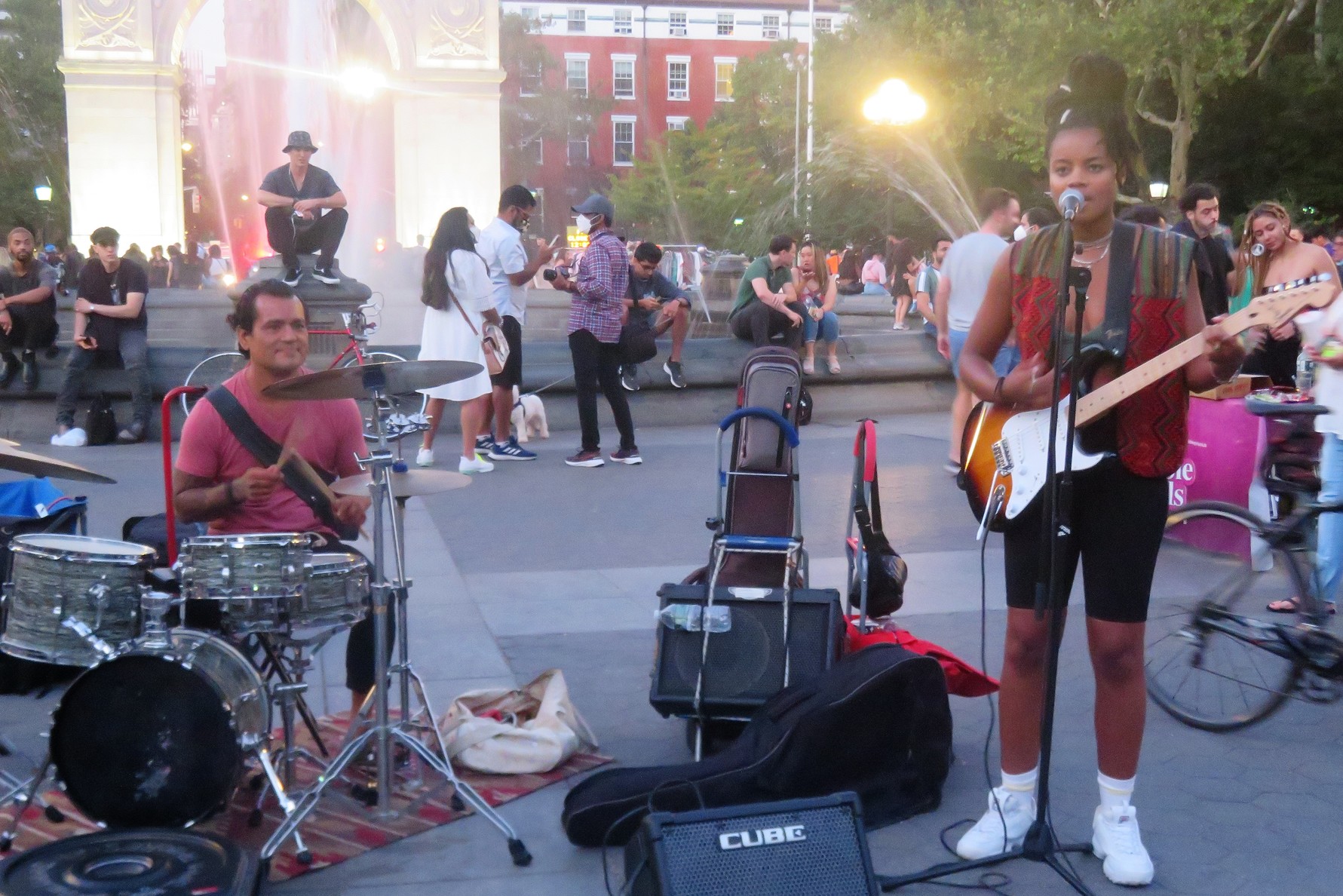This color photograph captures an outdoor evening scene transitioning into night. Streetlights begin to illuminate the setting, a lively park-like area with an open circular patio surrounded by greenery and buildings. In the foreground, an impromptu band performance features an African American woman singing and playing an electric guitar. She wears a red and green vest over black biker shorts, complemented by white tennis shoes and socks. Her hair is styled in an updo, and she sings into a microphone while standing near a Cube-branded amplifier and her guitar case.

To the left, a man in a red t-shirt sits behind a drum set on a small rug. His drum setup includes cymbals, adding rhythmic beats to the performance. Behind the musicians, various people, including someone perched atop a stone structure, walk around and enjoy the music. The background reveals a bustling scene with groups of people talking and a hint of a carnival or festival atmosphere.